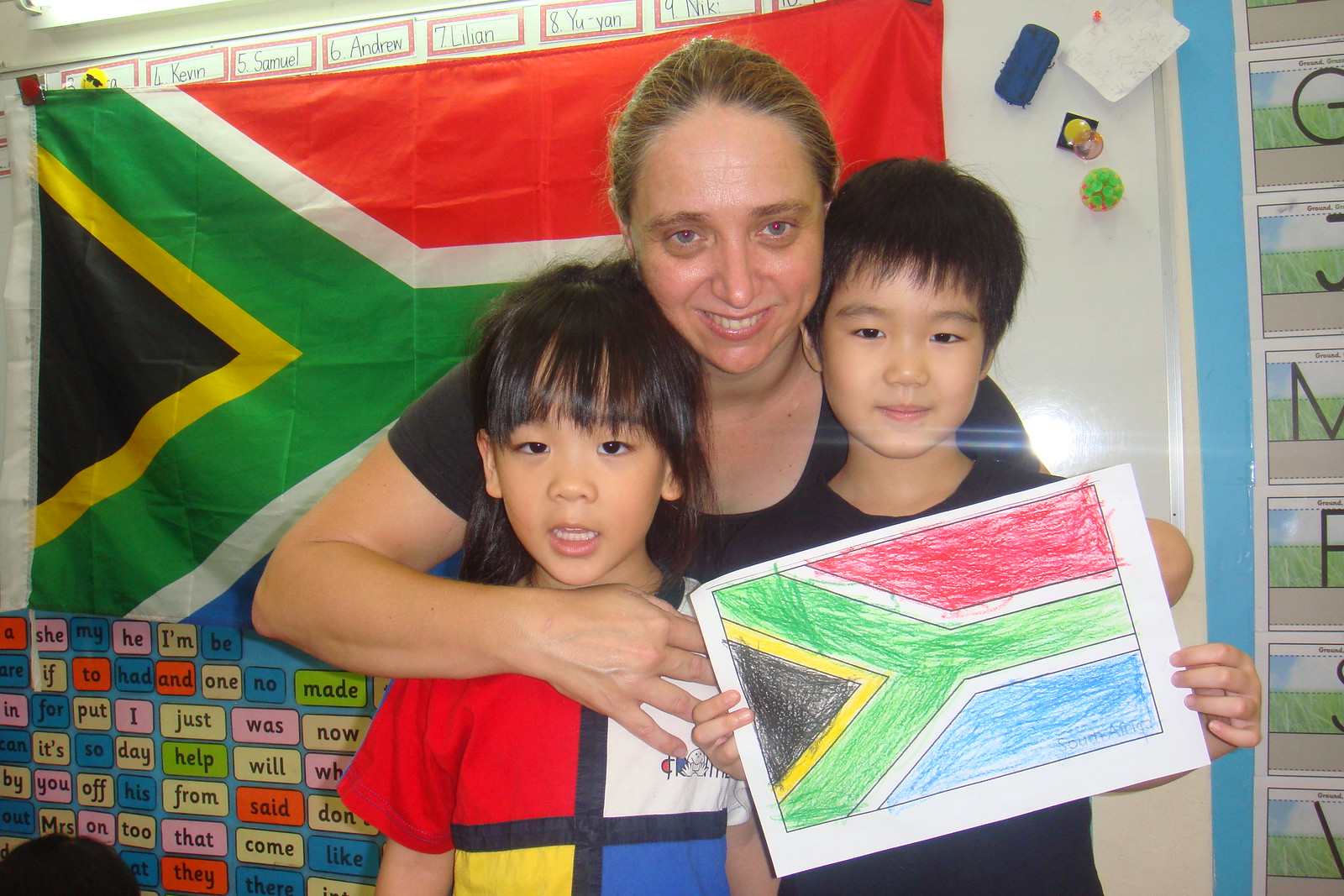In this image, we see a middle-aged woman with dirty blonde, light brown hair pulled back and light blue eyes, smiling and leaning towards the camera with her arms wrapped around two young Asian children. The woman, who appears to be in her late 30s or 40s, and the boy on the right are both wearing black t-shirts, while the little girl on the left is dressed in a shirt with red, blue, yellow, and white colors. Both children have dark hair and eyes. The boy on the right is holding a colored drawing of a distinct flag that matches a larger, actual flag displayed behind them on the wall, which features a black triangle with yellow outline, green design with white outline, red top, and blue bottom. Above the flag are rectangular papers with children's names bordered in red. The background suggests a classroom setting with small words on cards likely used to help children learn to read. The scene is cropped around the children's torsos, and there are magnets on the right side of the image.